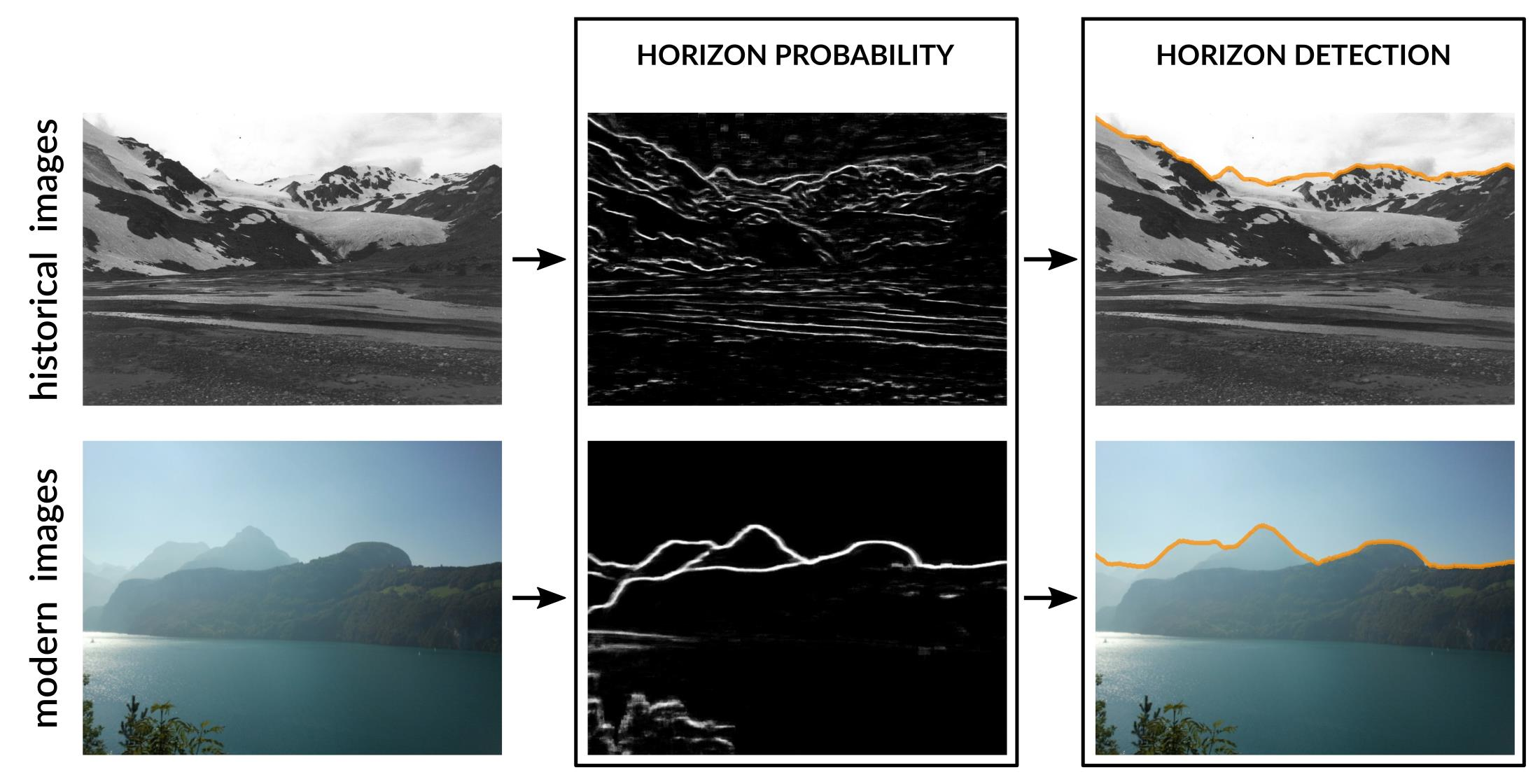The image consists of three columns featuring six pictures, two in each column. The leftmost column showcases "Historical Images" at the top with a black and white photo of a hillside, followed by "Modern Images" below it, depicting a lake with a mountain backdrop. Each of these landscape photos has an arrow pointing to the middle column, labeled "Horizon Probability." This column includes grayscale graphical representations of horizon probabilities for each corresponding image. Further arrows extend to the rightmost column, titled "Horizon Detection," where both the historical and modern images are re-displayed with a yellow line marking the detected horizon line. The historical image showcases a mountain horizon highlighted in yellow, while the modern image similarly features a yellow horizon line delineating the mountainous landscape.